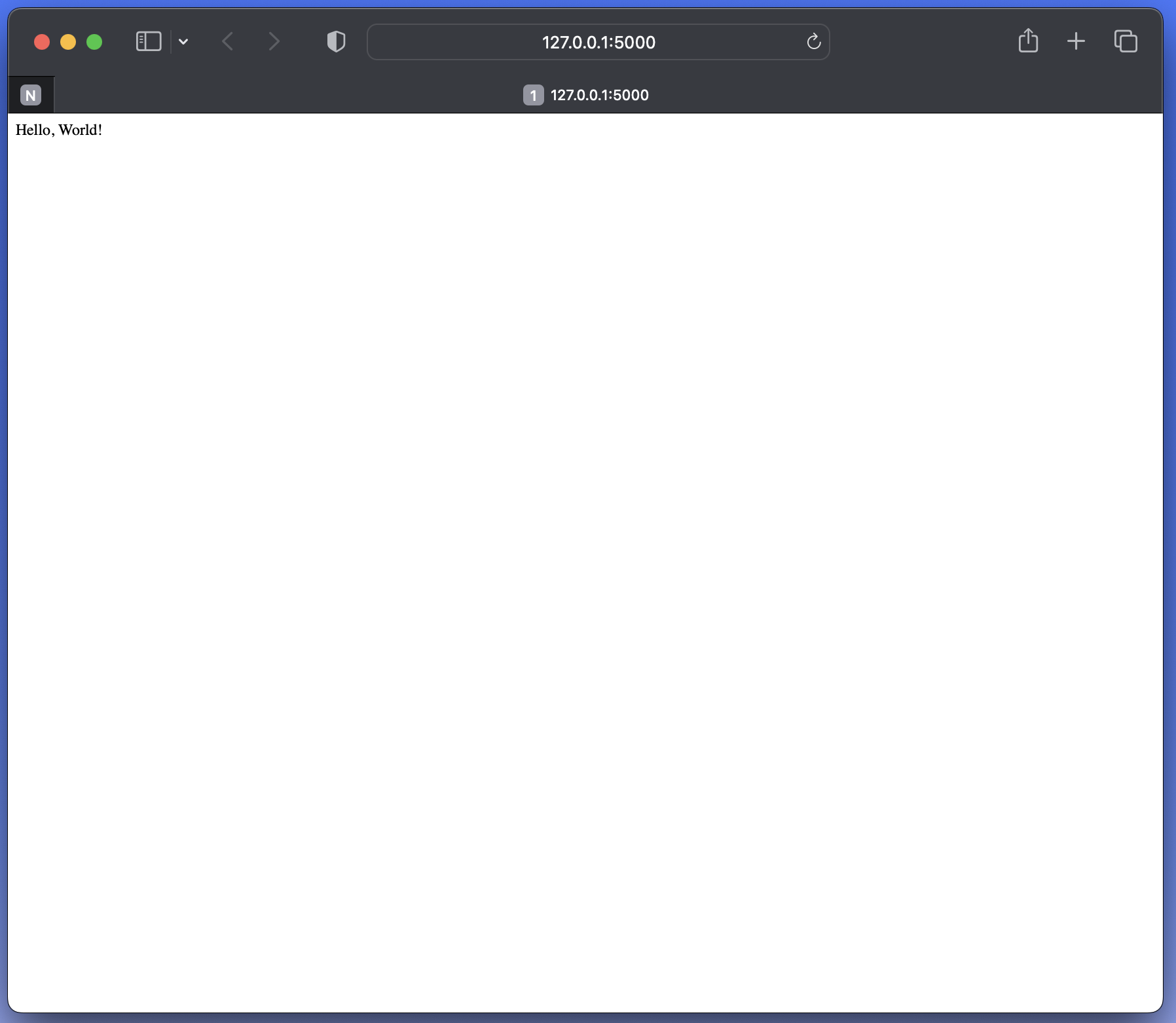Website Interface Description:

The website features a black navigation bar positioned at the top of the page, with distinct colorful accents on the left side in shades of red, orange, and green. Centrally located within this bar is a search bar displaying numbers. Flanking the search bar, both on the left and right, are various icons.

On the left side of the page under the black bar, there's a light gray box with a prominent "N" at its center, surrounded by a black border, and below it, some numerical information. Adjacent to this, there's a smaller gray box displaying the number "1".

Beneath these elements, a large white screen dominates the page with the text "Hello, World!" followed by an exclamation point. This white screen is devoid of any other content. The right side of this screen is bordered by a thick blue outline, while the left side features a thinner blue line. The blue outline at the top appears to balance between these two thicknesses. The bottom edge of the screen is distinguished by a black outline instead of blue.

The page is mostly blank aside from these elements. In the search bar, there's a distinct circular icon with an arrow, adding a touch of functionality to the minimalist layout.